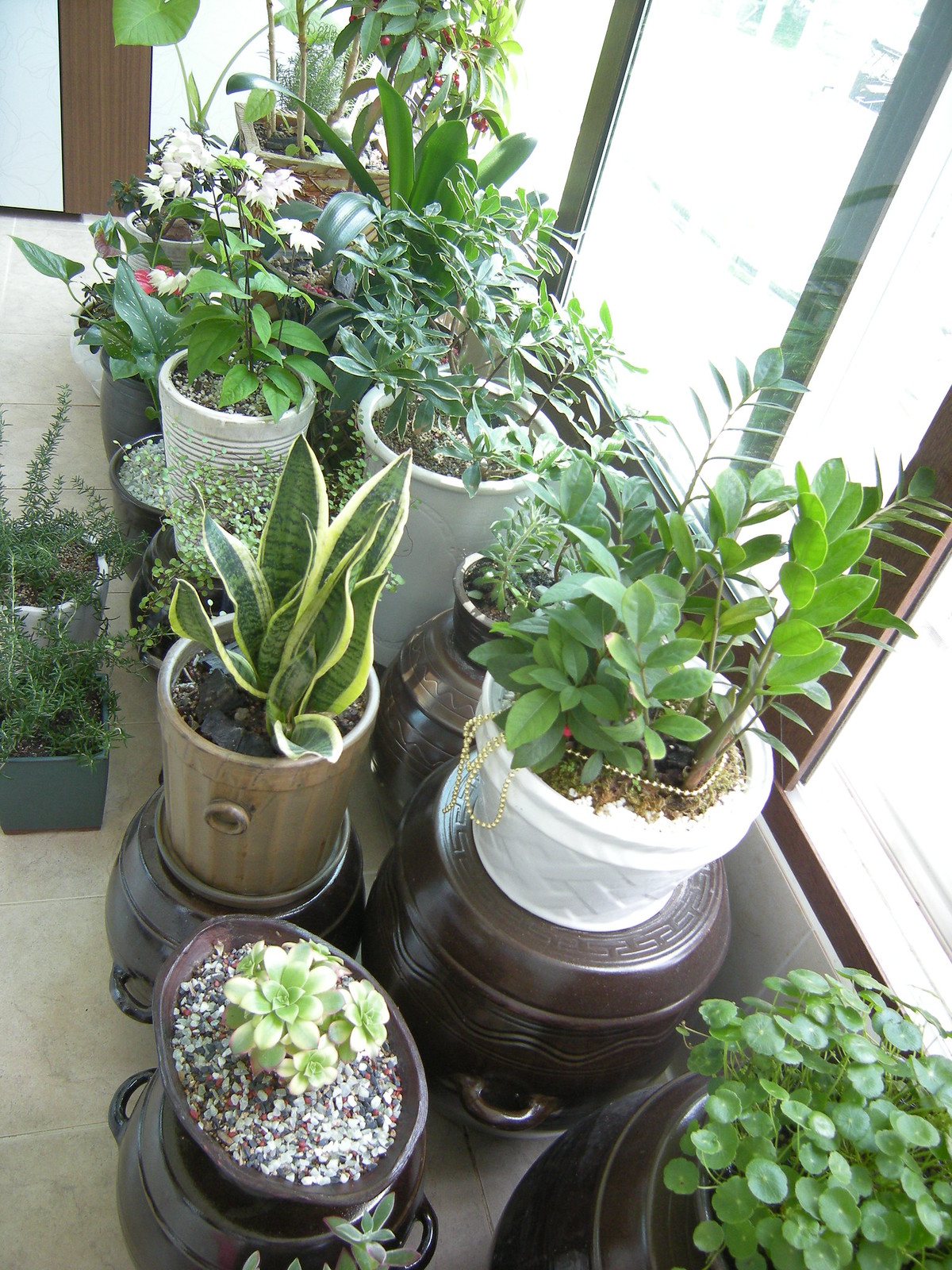The photograph captures an eclectic collection of potted plants arranged in a porch-like room bathed in natural light. The room features a light-colored tiled floor and a wall of multiple windows with wooden frames, providing ample illumination. The plants, varying greatly in type, size, and color, span the length of the windows, creating a lush green backdrop despite the diversity in individual plant appearances. 

Notable plants include a snake plant with tall, striking green leaves; another with spiky leaves and gold beading; and one with small red berries. The lower right corner features a clover-like plant in a large brown pot with a gray rim. Beside it, a succulent sits in an oval-shaped brown planter. There is also a cactus with pinkish flowers emerging from a pot filled with colorful rocks, including light gray, maroon, and dark blue stones.

The planters themselves are as varied as their occupants, including colors such as white, black, brown, and beige. Some are simple and plain, while others boast designs or patterns, like the large circular white pot with a crisscross pattern. Materials range from wooden and ceramic to metal, and they are both round and square in shape. Some pots contain additional elements like small stones, enhancing the visual texture of the display. Overall, the scene exudes a sense of vibrant diversity and tranquil natural beauty.